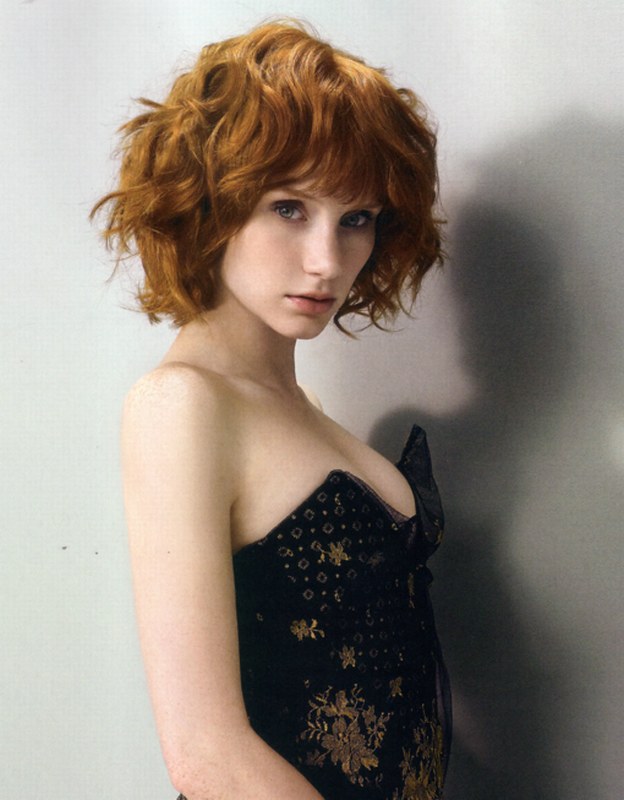The photograph captures Bryce Dallas Howard in a striking portrait against a solid light gray background. She stands in profile, slightly turning her head towards the camera, which emphasizes her solemn and serious expression. Her very fair, porcelain skin contrasts vividly with her vibrant red hair. The hair is wavy, cut in layers that create a shaggy, teased appearance, and it rests just below her chin, stopping above her shoulders.

Her piercing blue eyes and minimal, light makeup accentuate her natural beauty. Bryce's attire consists of a black sleeveless top with gold accents, featuring ornate beadwork or embroidery in floral and geometric patterns. The fitted top has a pronounced bust line that adds structure to her silhouette but does not complement her figure well. The image subtly conveys an air of sexual energy, highlighted by her poised stance and direct gaze into the camera. The overall composition is professional and crisp, with Bryce casting a subtle shadow on the wall behind her, adding depth to the image.